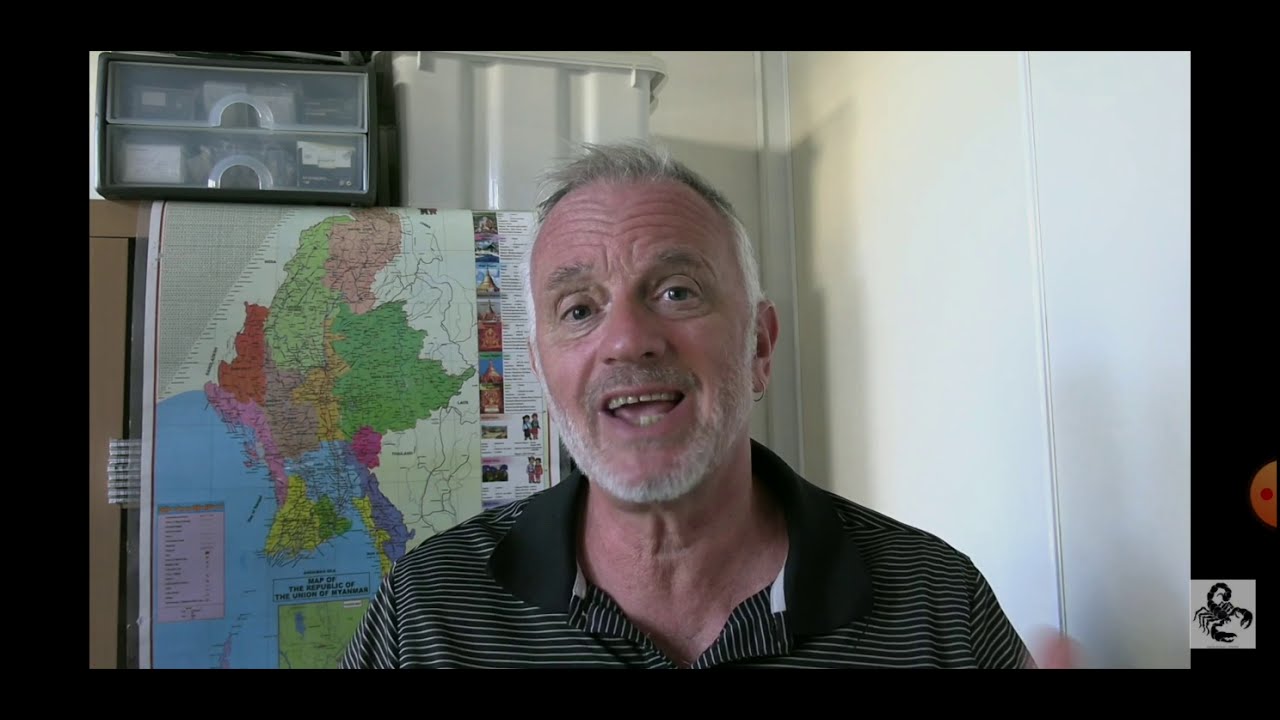The image is a screen capture, possibly from a Zoom call or online program, featuring an older man with a gray beard and mustache, and thinning gray hair. He is wearing a black and white horizontally striped polo shirt with a black collar and a few buttons unbuttoned. The setting is a white-walled room, and behind him on his right side is a colorful map with regions shaded in green, red, purple, blue, and yellow, bordered by a blue body of water. Above the map are small containers, including a two-drawer clear plastic one with a black frame and a white tote. The map appears to be attached to some shelving or a cabinet with a brown outer border. The image has a black border around it, and in the lower right corner, there is a small white square with a black scorpion logo. The man's mouth is open, suggesting he is speaking.